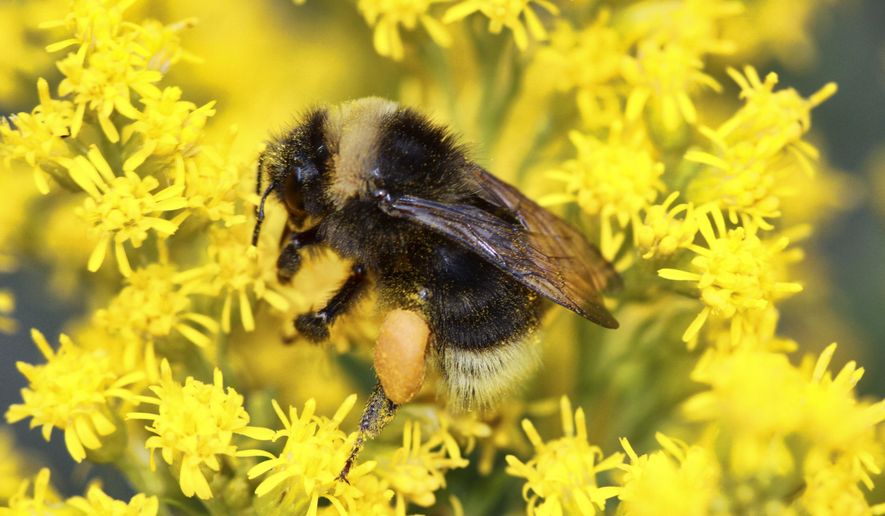This detailed image captures an outdoor scene focused closely on a bumblebee perched on a goldenrod plant. The bumblebee, with its yellow and black striped, fuzzy body, is prominently featured, showcasing its clear, slightly gray-tinted wings folded neatly on its back. The bee's yellow fuzz is evident on its head and tail, providing a striking contrast against its predominantly black fur. The image highlights a bulb of yellow pollen attached to the bee's back leg, demonstrating how it collects and stores pollen. The surrounding goldenrod flowers are a vibrant yellow, creating a picturesque background that fades into a soft, blurry focus, drawing attention to the crisp details of the bumblebee at the center.